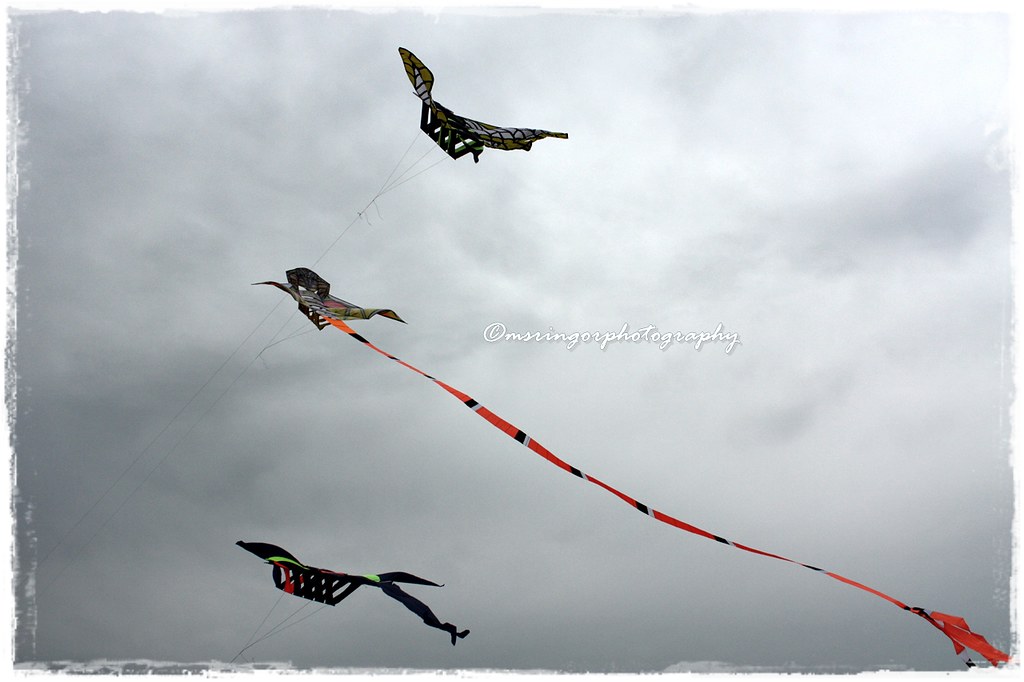In the picture, three distinct kites are soaring against a dark and cloudy gray sky. The kites are arranged vertically from bottom to top on the left side of the image, each one positioned slightly above the other. The kites exhibit a butterfly-like pattern, predominantly in black with accents of different colors. The bottom kite has a black base with green stripes at the top and red mixed in, and features two black ribbons on its right side. The middle kite is particularly striking with its long reddish-orange tail adorned with black and white stripes, adding to its thin appearance. The top kite, resembling the others with its butterfly-like wings, displays a mix of black and possibly yellow and white hues. All the kite strings trail towards the bottom left-hand side of the image. In the midst of the picture, there's a small logo or name of a photography company printed in cursive white text, blending subtly with the overcast background.